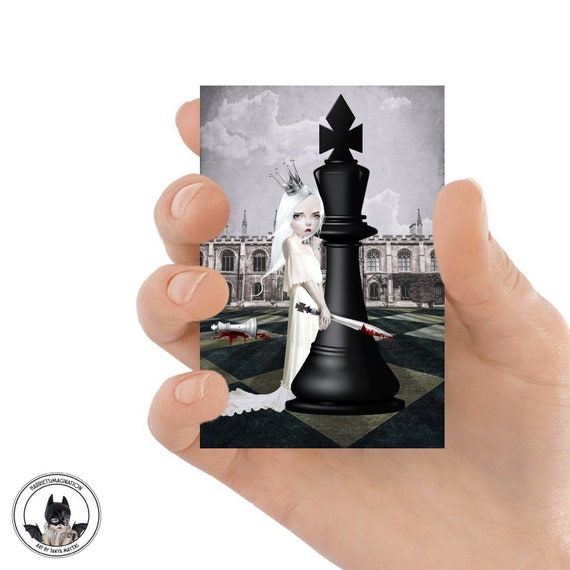In the image, a Caucasian hand devoid of nail polish holds up a card or a 4x6 picture, which appears to be an illustration. The focal point of the card features a white-haired girl, adorned with a silver crown, wearing a white dress cinched with a black belt. She holds a bloodied sword in her right hand and stands beside or clings to a large chess piece, either a king or queen. The background reveals a toppled white chess piece, spilling blood across the chessboard, and a European-style or Russian-like building under a cloudy, grey sky. The girl has a disgusted expression as she meets the viewer's gaze. Additional elements include a logo for branding or design at the bottom left, though it remains illegible.